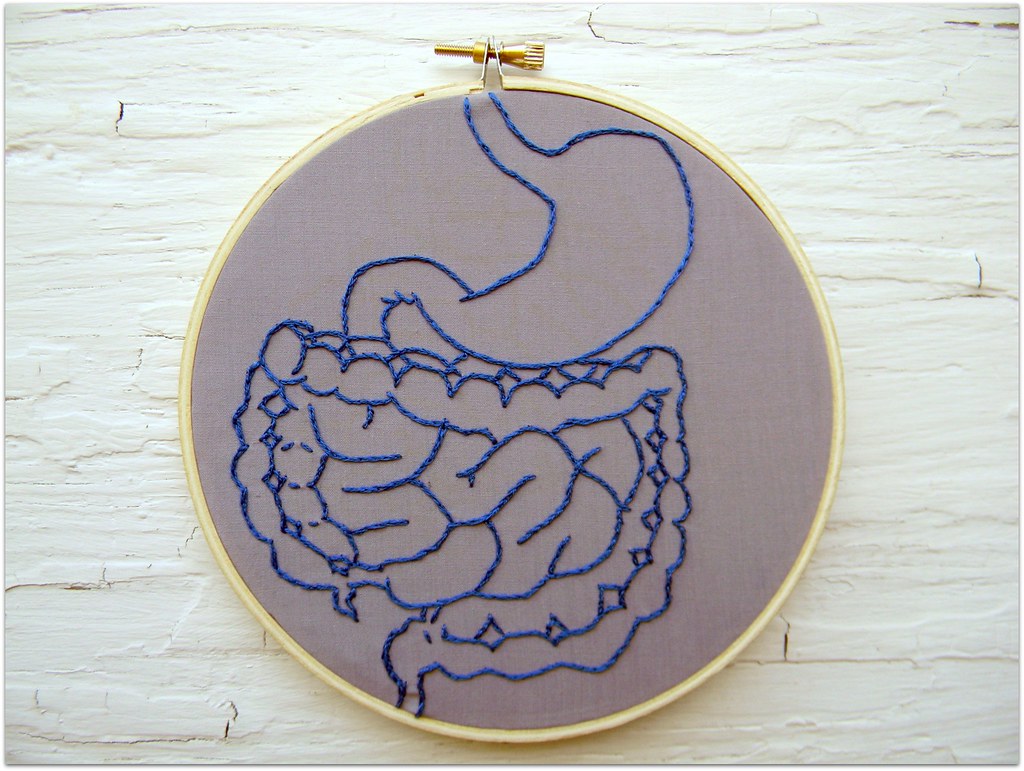This photograph showcases a detailed piece of fiber art encased in a circular wooden embroidery hoop, secured with a gold screw at the top. The fabric stretched within the hoop is a brownish-gray linen, creating a canvas for the artwork. The embroidery, executed entirely in royal blue thread, depicts an outline of the human digestive system, including the stomach, large intestine, small intestine, and descending to the colon area. The embroidery style is characterized by thick stitches, creating a textured effect with bumps, ridges, and squiggles to mimic the intricate details of the intestinal tract. The piece is slightly off-center within the hoop, and the background on which the hoop rests resembles a weathered surface with chippy white paint, possibly indicating an old painted wood or textured cement backdrop.